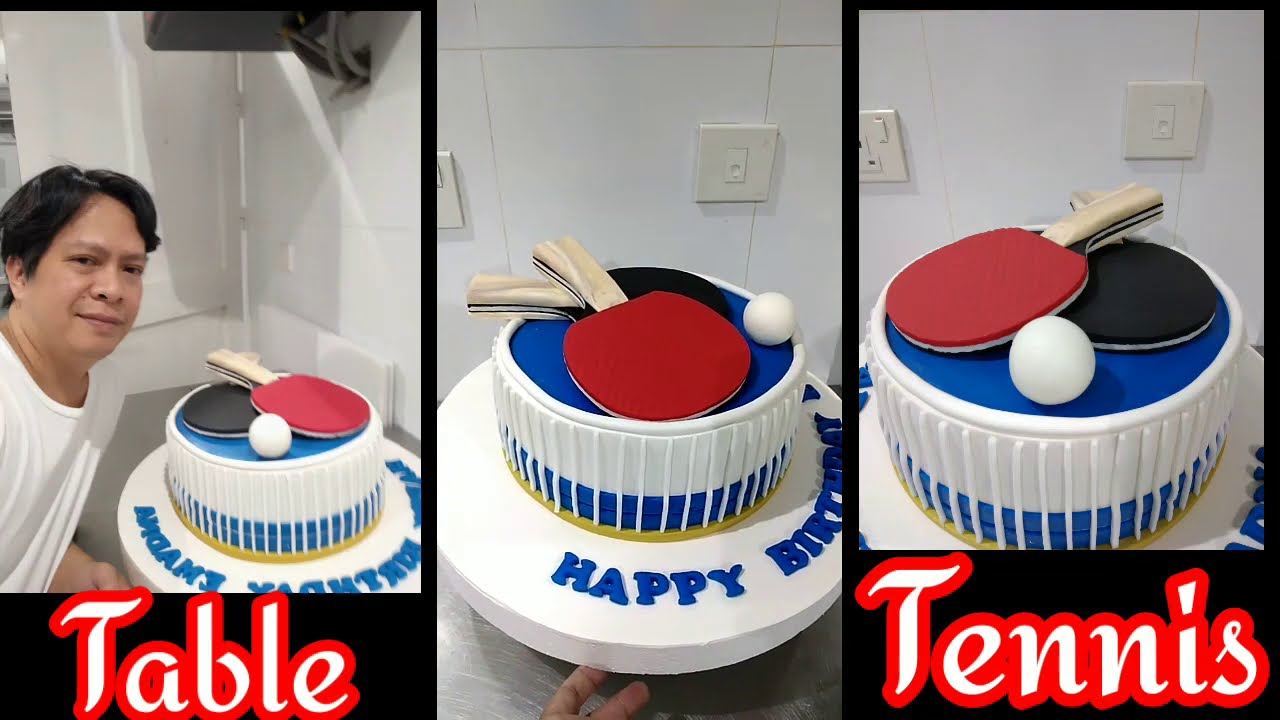The image is divided into three sections, each showing a different perspective of a table tennis-themed birthday cake. The left image features a man with black hair wearing a white t-shirt, who is slightly smiling and gazing at the cake, possibly the birthday celebrant or the baker. The middle image showcases the man holding or touching the cake with a couple of fingers, emphasizing the details on the cake's surface. The right image is a close-up of the cake's top. 

The cake itself is intricately designed with a white base, adorned with blue and very small yellow stripes around the bottom edge. Vertical white stripes run up and down the sides of the cake, creating a pleasing pattern. The top of the cake displays two table tennis paddles crossed—one red with a white handle on top of a black paddle with a white handle. A small white ping pong ball is positioned in front of the paddles. The cake sits on a larger white circular base with "Happy Birthday" written on it in blue frosting. Beneath the birthday message is the theme, "Table Tennis." 

The entire setup is located in what appears to be a white kitchen, adding a clean and crisp backdrop to the vivid colors of the cake.